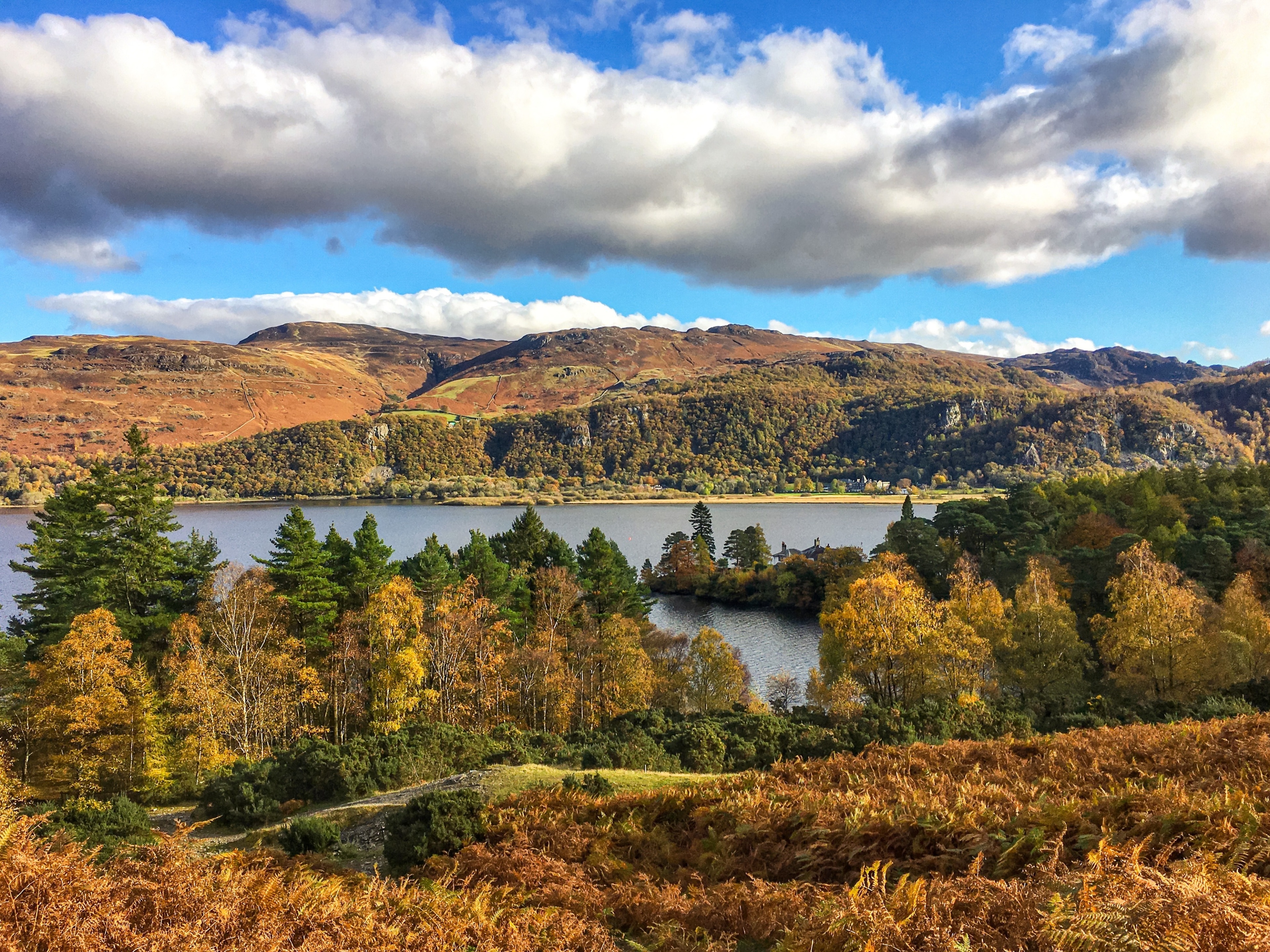This image captures a stunning autumnal mountain landscape bathed in clear, bright daylight. The top third of the photograph features a vibrant blue sky dotted with fluffy white and slightly gray-tinged clouds. In the background, a range of gently rolling, eroded mountains covered in thick forests stretches across the scene. The front face of the mountains displays rugged, boulder-strewn cliffs that descend towards a broad, placid river, hinting at a serene wilderness.

Golden-hued grasses and low shrubs dominate the immediate foreground, while further down the hill, a band of lush green foliage and tall trees—some evergreens and some deciduous turning shades of yellow—edge the river. The scene also includes a picturesque little peninsula jutting out into the calm river waters. While there are no people visible, hints of human presence are seen in the form of a few distant buildings on the far bank of the river, easily overlooked amidst the natural splendor. In parts of the foreground, a possible trail or road of gray gravel meanders through the vegetation towards the water, adding a subtle sense of depth and pathway in this pristine, peaceful landscape.